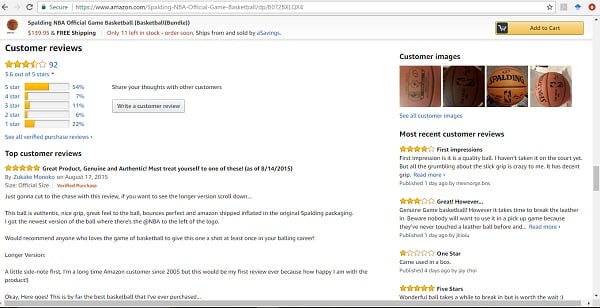This image displays the customer reviews section of the Amazon product page for the Spalding NBA Official Game Basketball. The item's listing indicates that it's available as a bundle, though the bundle details are not specified in the image. The price is slightly blurred but is noticeable as being over $100, and the listing highlights that free shipping is available. There are currently only 11 units in stock.

The basketball has an overall rating of 3.6 out of 5 stars, based on 92 customer reviews. The breakdown of ratings reveals that 54% of the reviewers awarded it 5 stars, 7% gave it 4 stars, 11% rated it 3 stars, 6% gave it 2 stars, and 22% assigned a 1-star rating. The image shows customer-uploaded photos of the basketball on the left side, alongside the top customer reviews.